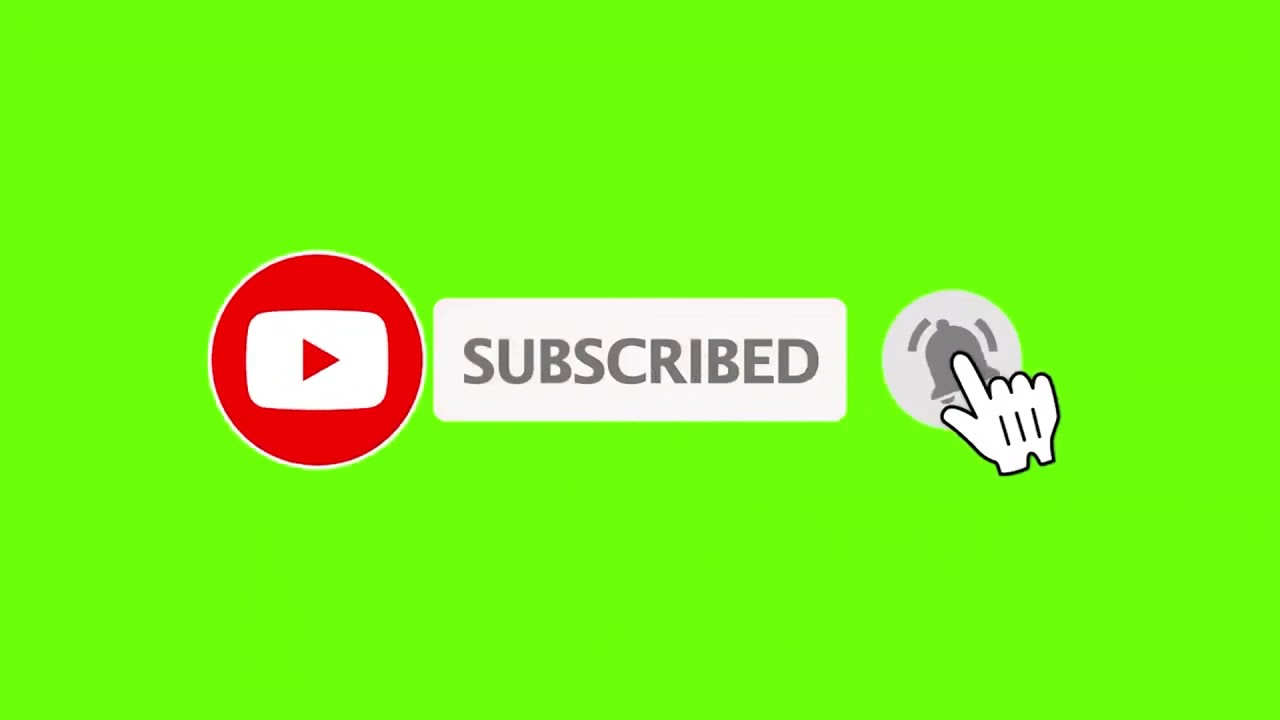The image features a vibrant neon green background. Centrally located on this bright backdrop, there are three distinct elements that together take up about a quarter of the total space: 

1. A red circle with the white YouTube logo in the form of a play button.
2. Immediately to the right of the YouTube logo is a rounded white rectangle with the word "Subscribed" written in gray font.
3. Further to the right, there is a light gray circle containing a gray bell icon. Overlapping the bell is a white, cartoonish hand with an extended index finger, pointing directly at the bell, giving the impression that the bell is ringing.  

All elements are aligned horizontally in the center of the image, which emphasizes the bright neon green background surrounding them.